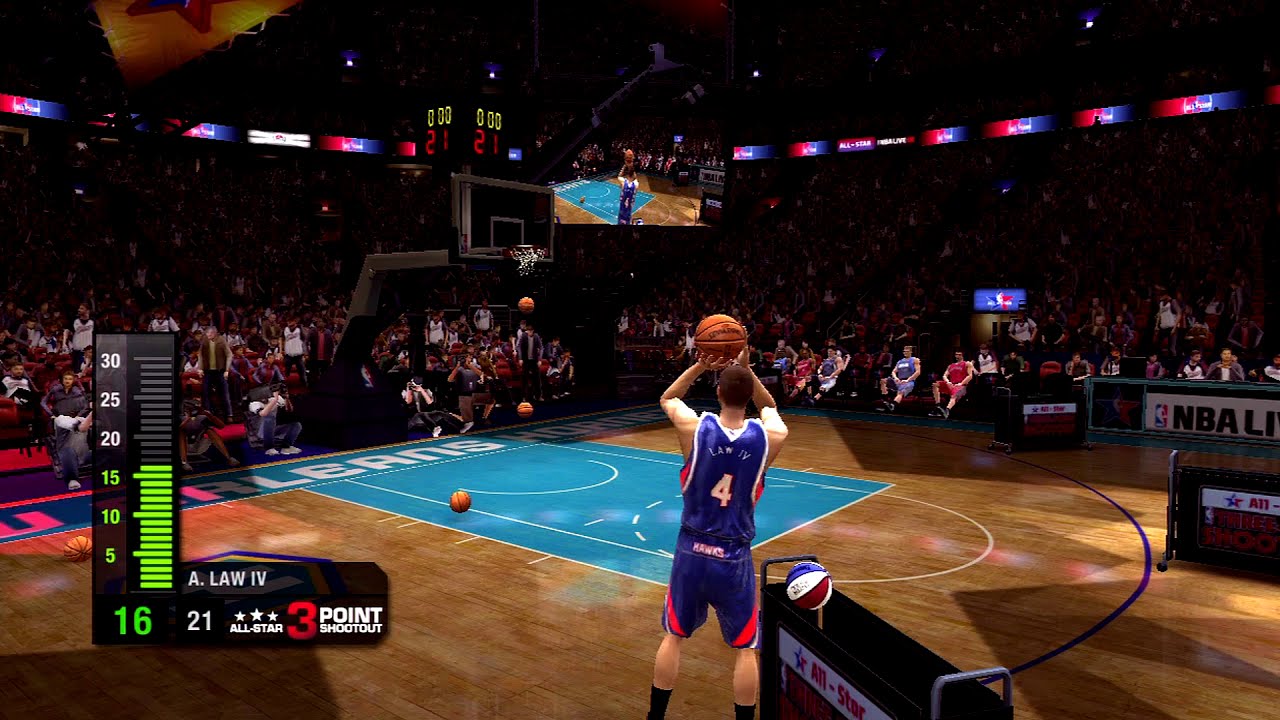The image is a detailed screenshot from a basketball video game, depicting a lifelike 3D model of a male player wearing a blue jersey with the number 4. The player's jersey and shorts feature a color scheme of red, white, blue, and a touch of black. He is in mid-air, preparing to shoot an orange-and-yellow Spalding basketball, aiming for a three-point shot. The player's figure dominates the center-bottom part of the image. In the foreground on the left, a ball rack with one remaining ball, matching the player's uniform colors, can be seen. The game's interface elements include a gauge at the bottom-left, reading 16. Behind the basketball hoop, an enthusiastic audience fills the stadium, with more spectators visible towards the right side and the back. The court segment visible is marked with a light blue rectangle near the goal area, adding to the immersive atmosphere of the game. A large TV screen in the corner allows the crowd to follow the action closely.